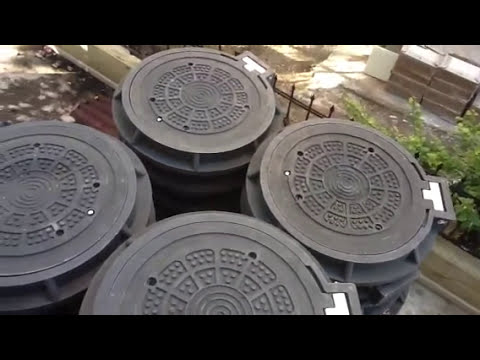The image depicts an outdoor industrial setting viewed from above, possibly taken with a drone. At the center, slightly towards the left, are four large, circular containers or lids that resemble manhole covers, each with a dark gray circular grid cover and a white hinge on the right side. These objects are stacked closely together, filling the vertical space of the image. They are situated in a yard with a lot of dirt, stonework, and brickwork, surrounded by a wrought iron fence in the background. The top right features some plants, indicating a mix of natural and industrial elements. The colors in the scene include tones of gray, brown, white, green, yellow, and tan. There is no text visible in the photograph, and the time appears to be mid-day, emphasizing a clear, detailed industrial realism style.